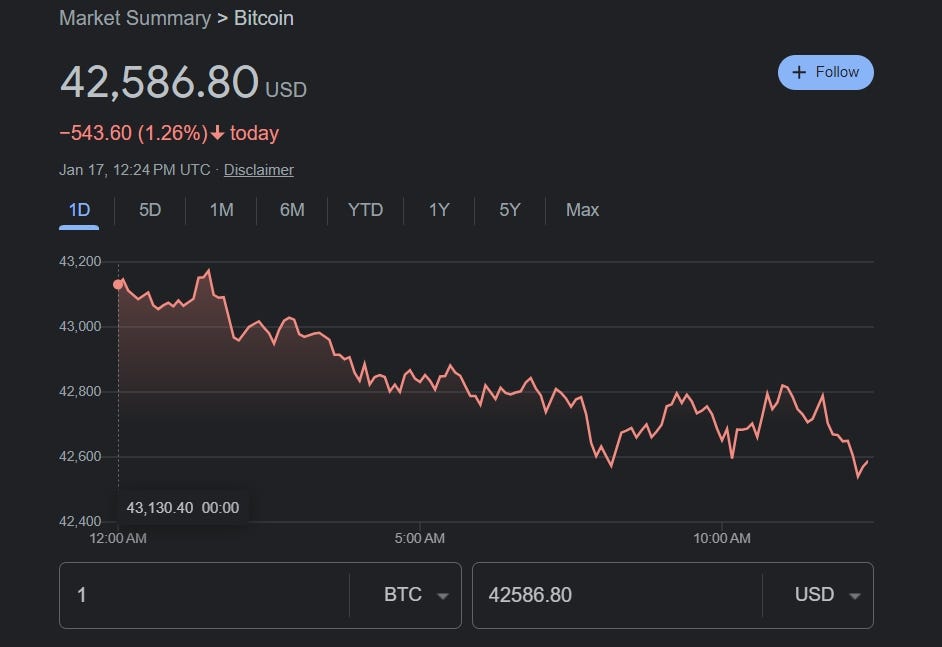This image is a screenshot displayed in landscape mode, featuring a black background. In the upper left-hand corner, there is a header that reads "Market Summary," followed by an arrow pointing to the word "Bitcoin." Below this, the current value of Bitcoin is listed as "$42,586.80 USD." On the right side of this header, there is a light blue button labeled "Follow."

The next row is highlighted in pink, showing a negative change of "$543.60 (1.26% down) from the previous hour on January 17th at 12:24 p.m." Below this information, an underlined disclaimer is present.

Dominating the rest of the image is a chart depicting Bitcoin's price movements over the course of the day. At the bottom left, there are two drop-down menus – the first one displays "1 BTC," while the second one mirrors the current price "$42,586.80 USD."

The chart illustrates a decline in Bitcoin's value, starting from approximately $43,000 at midnight and descending to the current price. The vertical axis on the left side of the chart is marked with gridlines at intervals of $42,400, $42,600, $42,800, $43,000, and $43,200. The horizontal axis along the bottom is labeled with time stamps at 12 a.m., 5 a.m., and 10 a.m. The price trend line shows minor fluctuations but overall indicates a downward trajectory.